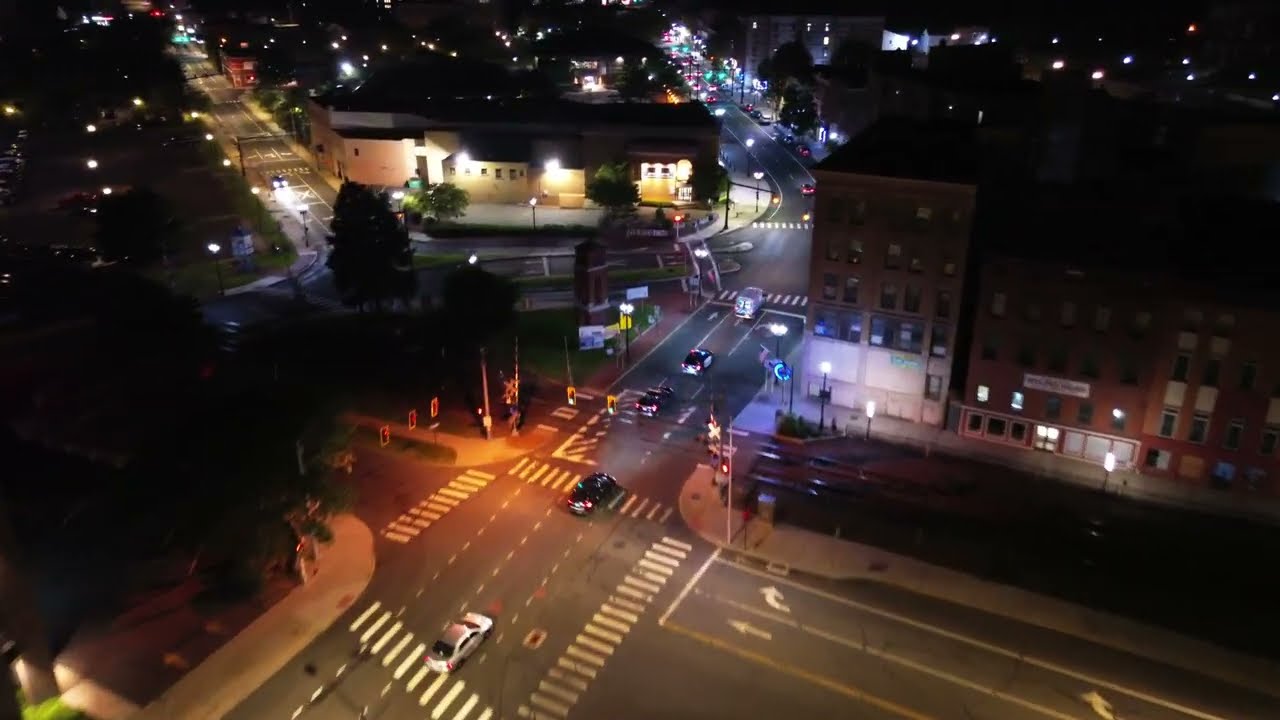This image presents a detailed overhead view of a bustling city intersection at night, illuminated by an array of street lights and vehicles' headlights. The intersection, which likely serves as a core junction in the city, features prominently marked white-striped crosswalks and directional arrows pointing straight, left, and right. Several vehicles occupy the streets, either in transit or recently having passed through. Sodium vapor street lamps cast a warm glow over the asphalt, while neon lights from nearby storefronts add splashes of color to the scene.

In the bottom right of the image stands a five-story building that exudes a warehouse-like appearance, though it could also house apartments or shops, particularly on the lower floors. Adjacent to this building, to the left, stretches a dark, tree-lined area suggesting the presence of a park or green space that contrasts with the bright urban surroundings.

Towards the top of the image, the road curves to the left, illuminated by more streetlights and lined with additional vehicles waiting at another set of traffic lights. This section features more buildings, both commercial and possibly residential, as well as another stretch of greenery. A small triangular area, possibly a mini-park or plaza, is nestled among the thoroughfare, adding a touch of nature to the urban environment. The entire scene, with its array of buildings, bustling cars, and varying light sources, encapsulates the vibrant yet intricate essence of city life at night.